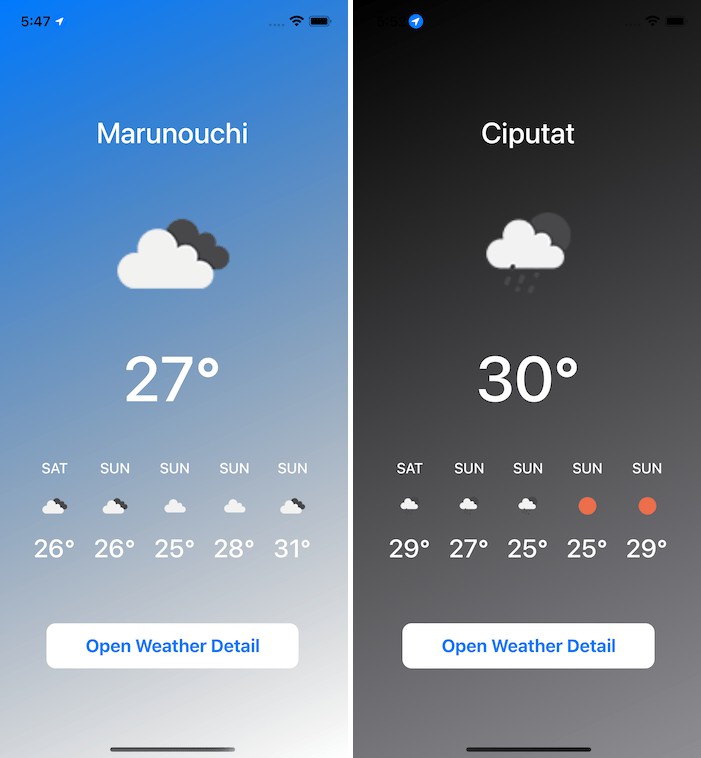Here is a cleaned and detailed version of the caption:

---

The image displays a weather forecast for Marunouchi, featuring a detailed layout. At the top, a blue circle indicates full Wi-Fi and battery connectivity, symbolized by four bars each. Below this, various clouds and temperature readings are arranged in a sequence. 

- Saturday: A grey cloud icon with 27°C.
- Sunday: A grey cloud icon with an initial reading of 26°C and later updated to 35°C, then showing fluctuations at 20°C and 31°C.

Additionally, the forecast repeatedly references "Sunday" with temperatures adjusted to 20°C, 27°C, 25°C (twice), and 29°C. An option to "Open Weather Detail" is noted twice with a white rectangle and a line beneath it. The background shifts between grey and black elements, providing a visual contrast in the display.

---

Is there anything else you'd like to improve or any other assistance you need?